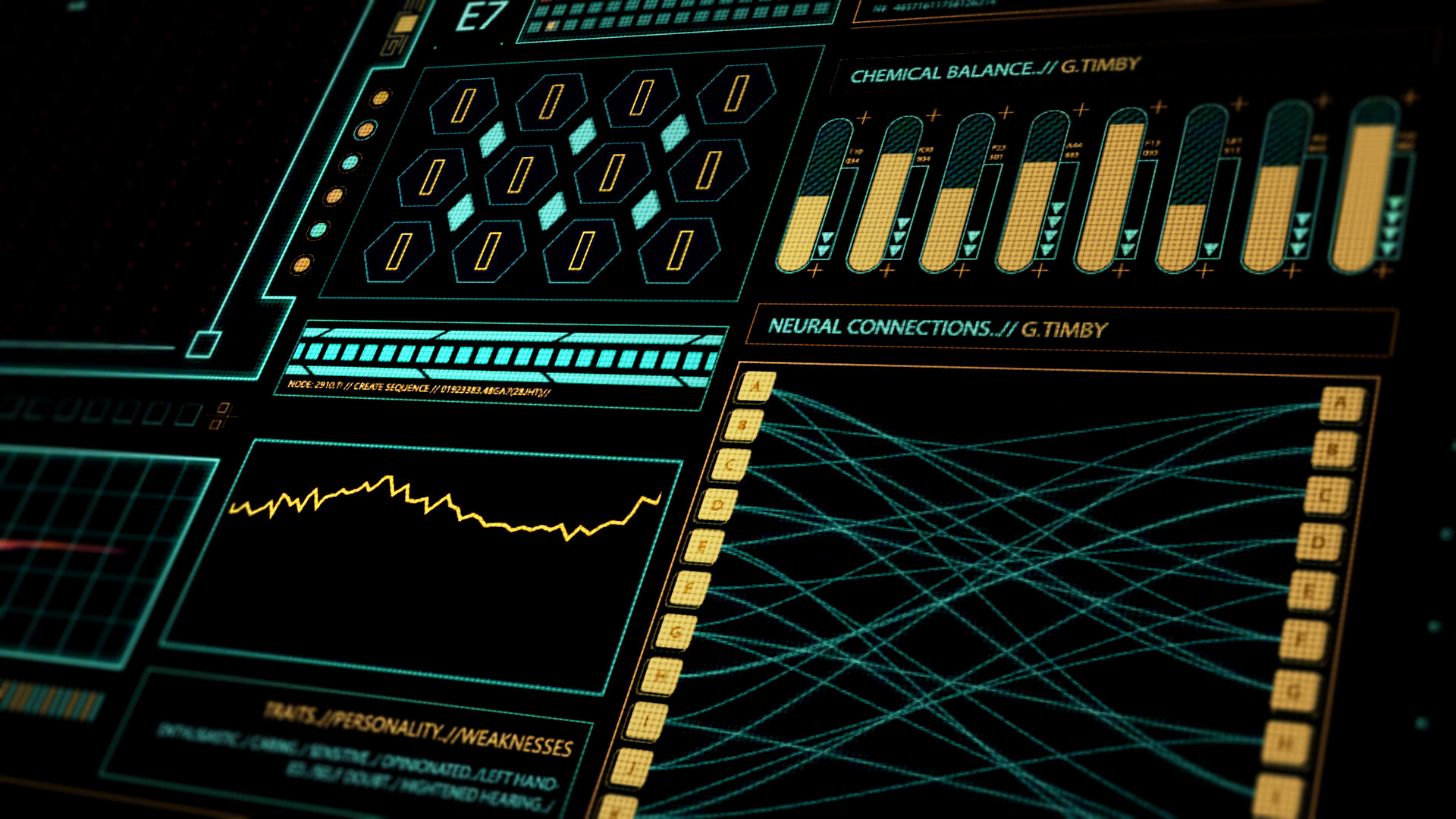The image is a detailed, futuristic user interface displayed on a black background. Predominantly using cyan and goldish yellow colors, it contains various graphs and charts labeled with technical headers such as "Neural Connections" and "Chemical Balance," both highlighted in blue. The "Chemical Balance" section, located at the top right, features multiple drawings of rounded rectangles resembling test tubes. These test tubes are light green with varying levels of yellow inside, representing different measurements.

Underneath this section, the "Neural Connections" area displays a structured chart with tiny yellow squares aligned on both the left and right sides. Lines emanate from these squares, creating a complex connection map. Below this, a line graph occupies the bottom left corner of the interface.

Additional textual data appears across the screen, including detailed readouts such as "node 2910.T1 // create sequence // 019233B3.48GA7," with further details enclosed in parentheses. At the bottom, labels such as "traits, personality, and weaknesses" provide further context, reinforcing the theory that this could be an advanced medical or perhaps even a quantum computer interface. The overall design exudes a high-tech atmosphere, suggesting its application in a cutting-edge field.